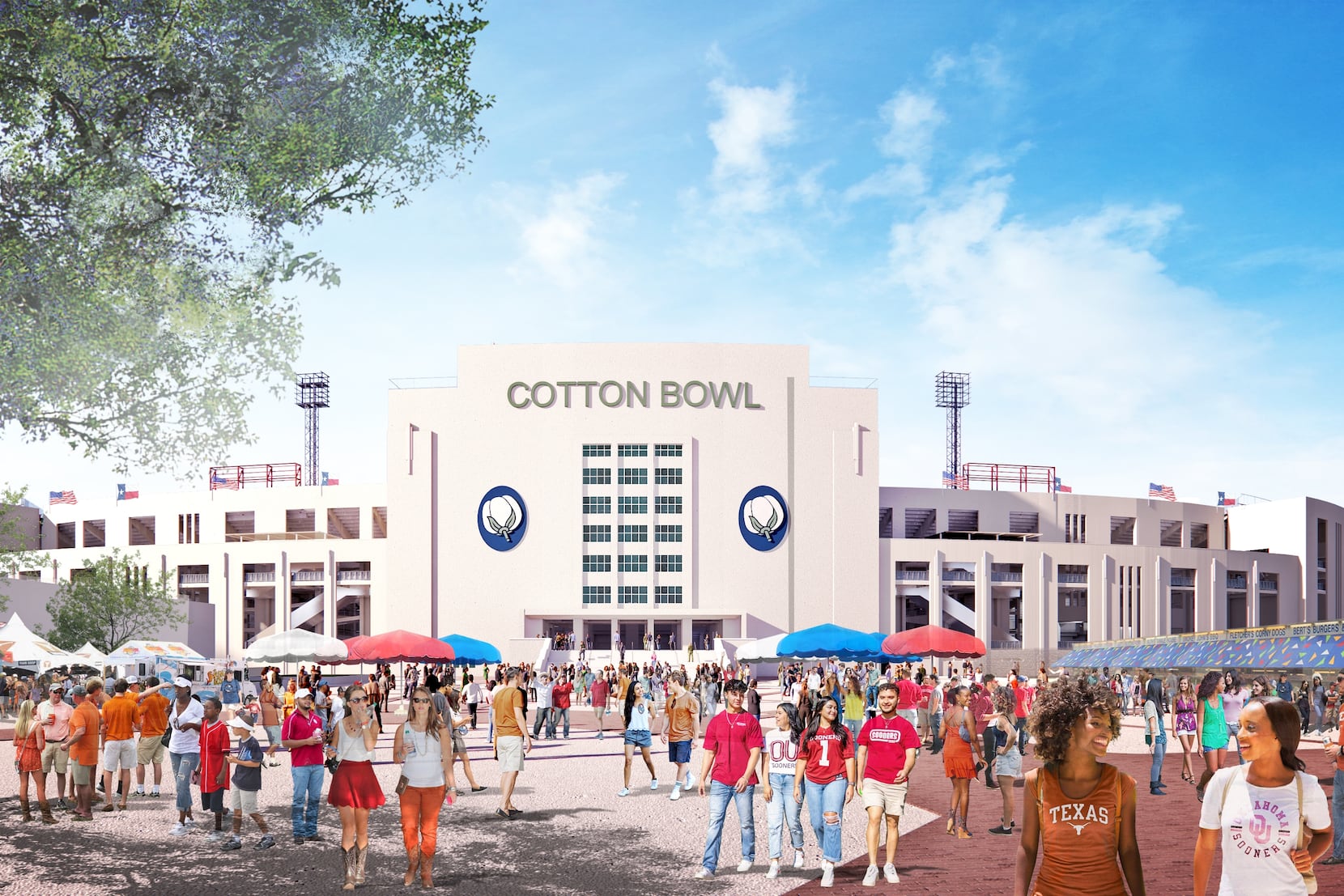The image captures a bustling outdoor scene during the day, centered on a grand, white Cotton Bowl stadium. The sky above is a vibrant blue with wisps of white clouds and a light haze toward the horizon. A green tree branches into the top left corner of the image, adding a touch of nature to the scene. Prominent on the building's façade, the bold black letters spell out "Cotton Bowl," flanked by two blue circles with white cotton bud images. The stadium's structure features a taller central section and stretches out into lower wings on each side, with five rows of windows enhancing its facade and a set of stairs leading up to the entrance.

In the foreground, a diverse crowd of people fills the scene, some wearing short sleeves, others in a mix of shorts and long pants, reflecting the casual, summery atmosphere. Many are gathered under large white, red, and blue umbrellas peppered throughout the area. Noteworthy in the crowd are several clusters: the bottom left features individuals in orange shirts, while the center-right has groups in red shirts, indicating possible team affiliations. Particularly eye-catching are two African American women at the bottom right corner, engaged in an enthusiastic conversation; one sports a brown shirt with 'Texas' emblazoned in white, and the other wears a white shirt partially obscured by sunlight. Overall, the scene combines architectural grandeur with the vibrant energy of the gathered crowd.